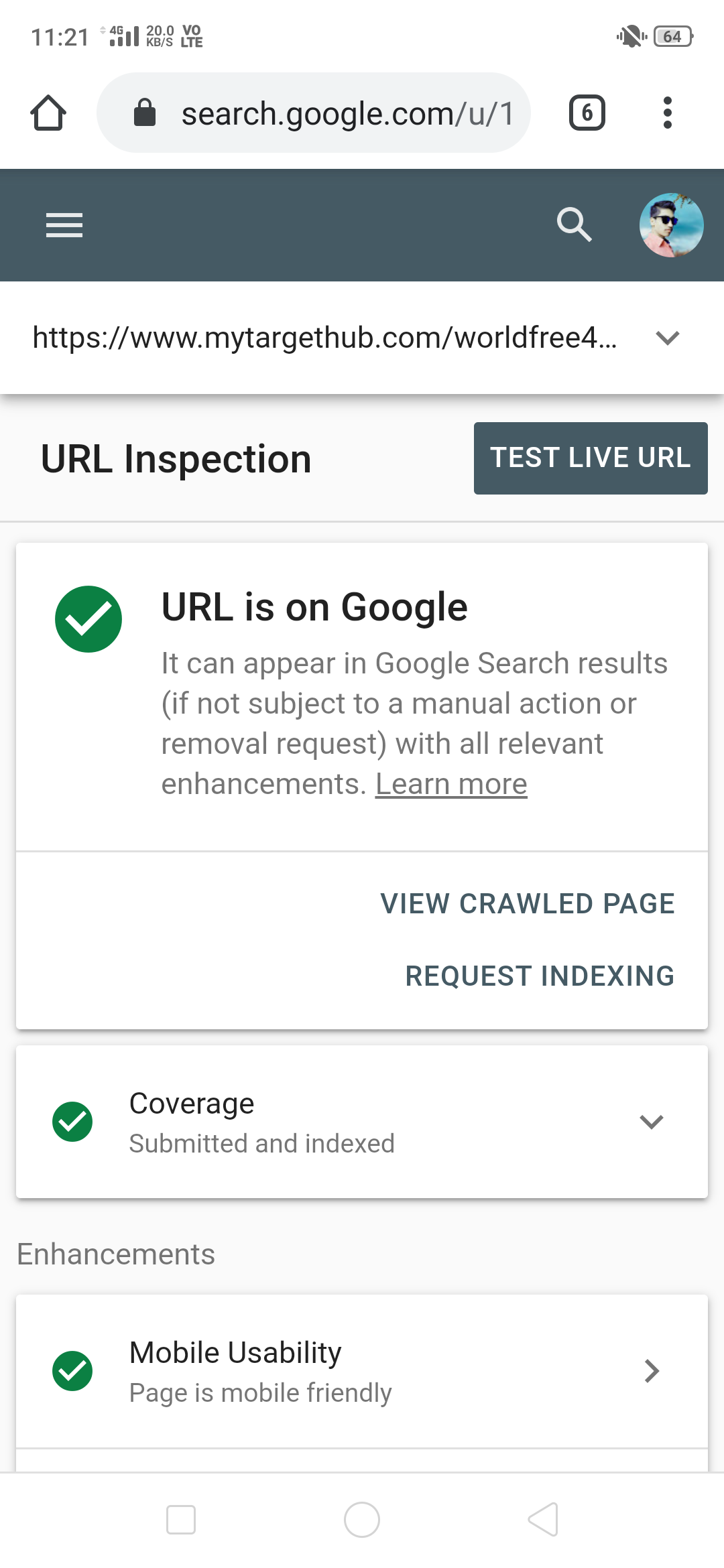This is a screenshot of a mobile phone displaying a web page from "search.google.com/u/one." The highlighted URL, "mytargethub.com," is visible, indicating the site in question. 

In the image, a man with short black hair, wearing a red shirt and sunglasses, is visible, enjoying a bright, sunny day. 

The main content displayed is a URL inspection report. "URL inspection" is prominently displayed in bold black letters, followed by a gray box containing white text that reads "Test Live URL." Below this, a green circle with a checkmark indicates "URL is on Google" in bold black letters. The subsequent smaller text clarifies that the URL can appear in Google search results unless subject to manual action or removal requests and includes relevant enhancements.

A faint gray line separates this from additional options: "View Crawled Page" and "Request Indexing." Beneath another subject heading, a green circle with a checkmark shows "Coverage Submitted and Indexed." The final subject addressed is "Enhancements," with an emphasis on mobile usability, denoted by another green circle with a checkmark and the statement "Page is mobile friendly."